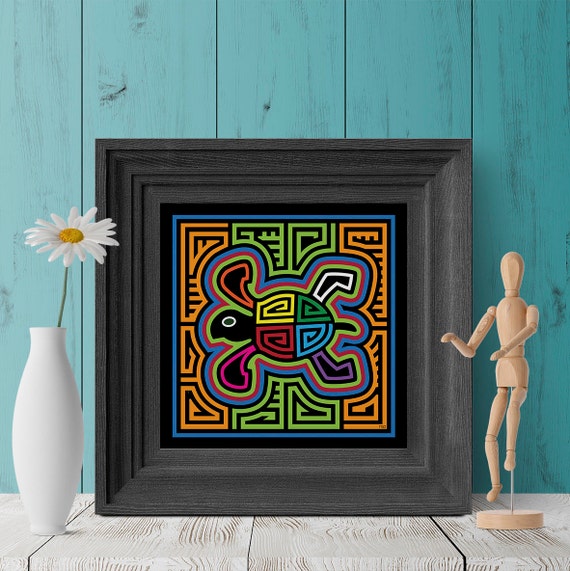In the photograph, a framed piece of multicolored stylized artwork depicting a turtle sits on a whitewashed wooden table, set against a blue-washed wooden wall. The dark gray wooden frame encloses a picture of a turtle composed of various geometric shapes and vibrant colors, including yellow, green, red, blue, and accents of orange. The turtle has a black head with a white-outlined eye. To the left of the framed art is a white, curvy vase showcasing a single white daisy. To the right, a wooden artist's mannequin, posed with its arms extended and right hand bent, adds to the creative ambiance. The arrangement sits harmoniously on the pale white wooden surface, offering a serene and artistic vignette.